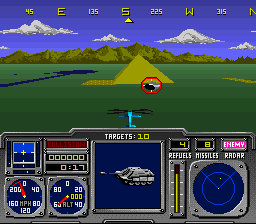The image is a highly pixelated screenshot of a retro video game, reminiscent of an Atari game from the 1980s. At the top of the image, a blue sky is dotted with white and gray clouds, overlayed with a series of yellow alphanumeric characters that include "40 45 E" and "225 W." 

Below the sky, there are dark brown and light brown mountains, with a green grassy field in the foreground. Centrally positioned in the field is a yellow, pyramid-like structure, resembling an Egyptian pyramid. There is a yellow circle with crosshairs overlaying part of the pyramid, likely indicating a target or point of interest in the game.

The bottom third of the image is dominated by the game's control panels. These panels feature a dark blue rectangle at the center, filled with numerous metallic and robotic elements, dials, and gauges. To the right, a circular blue clock-like gauge is prominent, while various controllers and displays with blue, black, yellow, and red stripes and white numbers fill the rest of the space. The text "Targets: 10" is visible, emphasizing the game's objective.